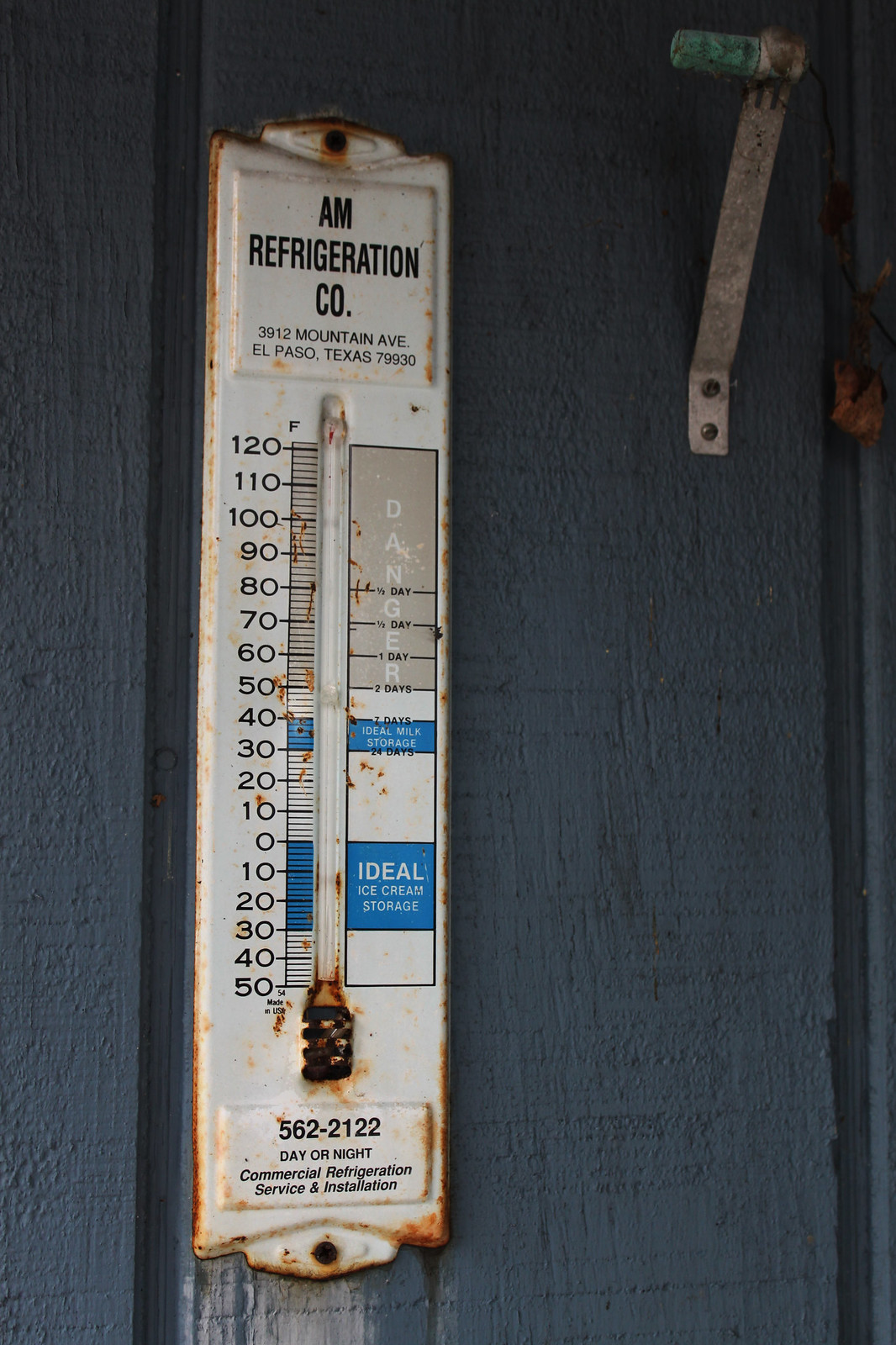This image depicts an old, vintage outdoor thermometer that is no longer functional due to severe rust. The thermometer, originally white, has been largely overtaken by rust, transforming the glass tube that once held mercury or its modern equivalent into a mere rusty pit. At the top of the thermometer, it is labeled "AM Refrigeration Co." and below that, in smaller font, the address "3912 Mountain Ave., El Paso, Texas, 79930" is printed. 

The thermometer has distinct sections highlighted in blue, indicating various temperature zones and their uses. The range from 0 to -30 degrees Fahrenheit is marked as "Ideal Ice Cream Storage," while 30 to 40 degrees Fahrenheit is labeled as "Ideal Milk Storage." Additionally, it specifies storage durations: "Seven days at 40°F, 24 days at 30°F." 

Between 50 degrees Fahrenheit up to an extreme of 120 degrees Fahrenheit, the range is marked with caution as "Danger." Within this range, various durations are listed: "52 days" possibly for 50°F, "61 days" for 60°F, "70" for a yet unspecified duration, and "half a day" for both 80°F and 90°F. 

At the bottom, the text reads "562-2122, day or night commercial refrigeration service and installation," providing contact information for services offered. The significant rust and wear suggest that this thermometer has been exposed to outdoor elements for a long time.